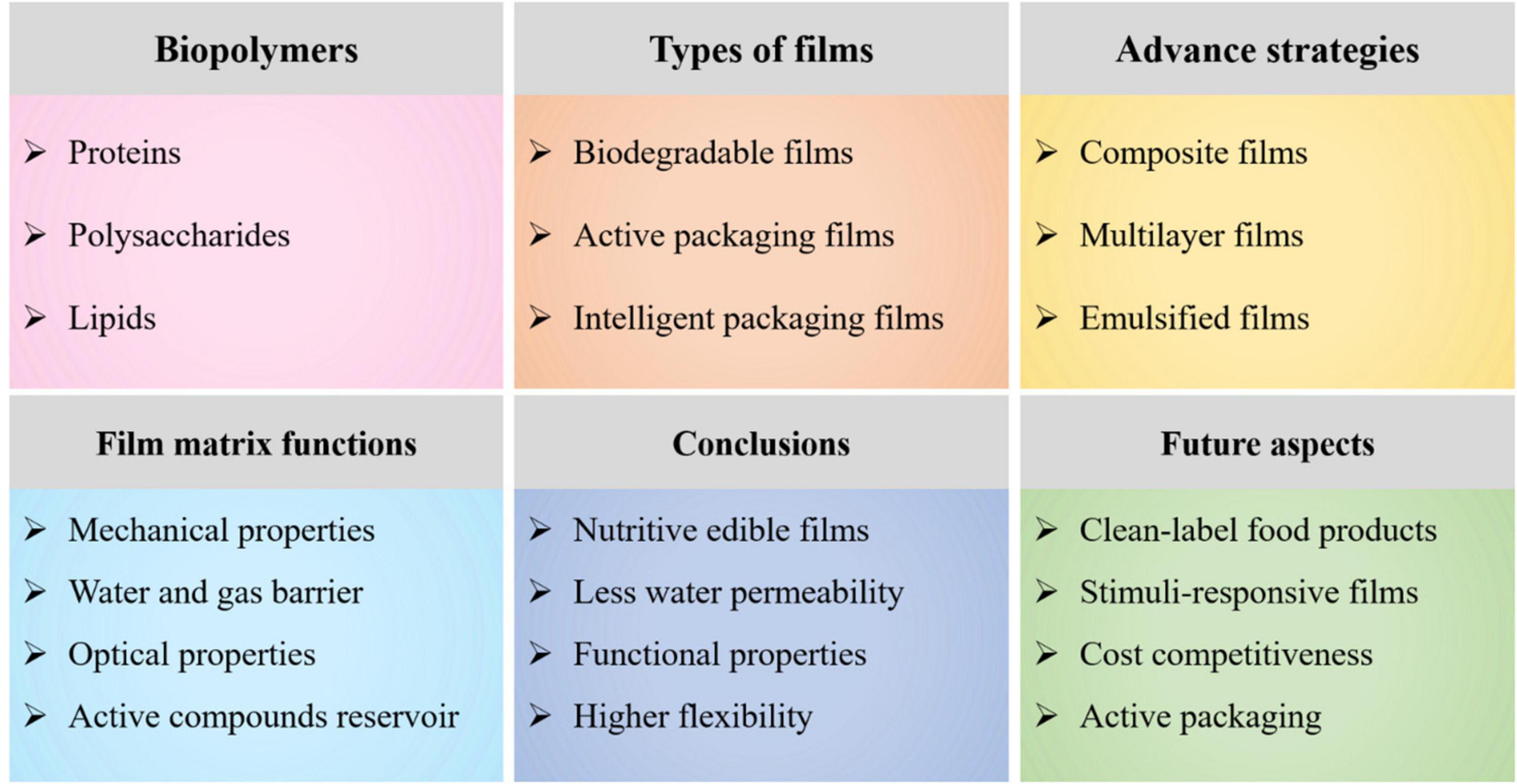The image depicts a detailed chart with six distinct, brightly colored sections, each representing key topics in the study of films and biopolymers. The first section, labeled "Biopolymers," is shaded in pink and lists proteins, polysaccharides, and lipids. The second section, "Types of Films," is orange and includes biodegradable films, active packaging films, and intelligent packaging films. The third section, "Advanced Strategies," is yellow and details composite films, multilayer films, and emulsified films. On the lower row, the fourth section, "Film Matrix Functions," is light blue, covering mechanical properties, water and gas barrier, optical properties, and active compounds reservoir. The fifth section, labeled "Conclusions" and colored bluish purple, mentions nutritive edible films, less water permeability, functional properties, and higher flexibility. The final green section, "Future Aspects," discusses clean label food products, stimuli-responsive films, cost competitiveness, and active packaging. Each section is distinctive with bold black font and aligned within the same structured layout, providing a comprehensive overview of the topics.